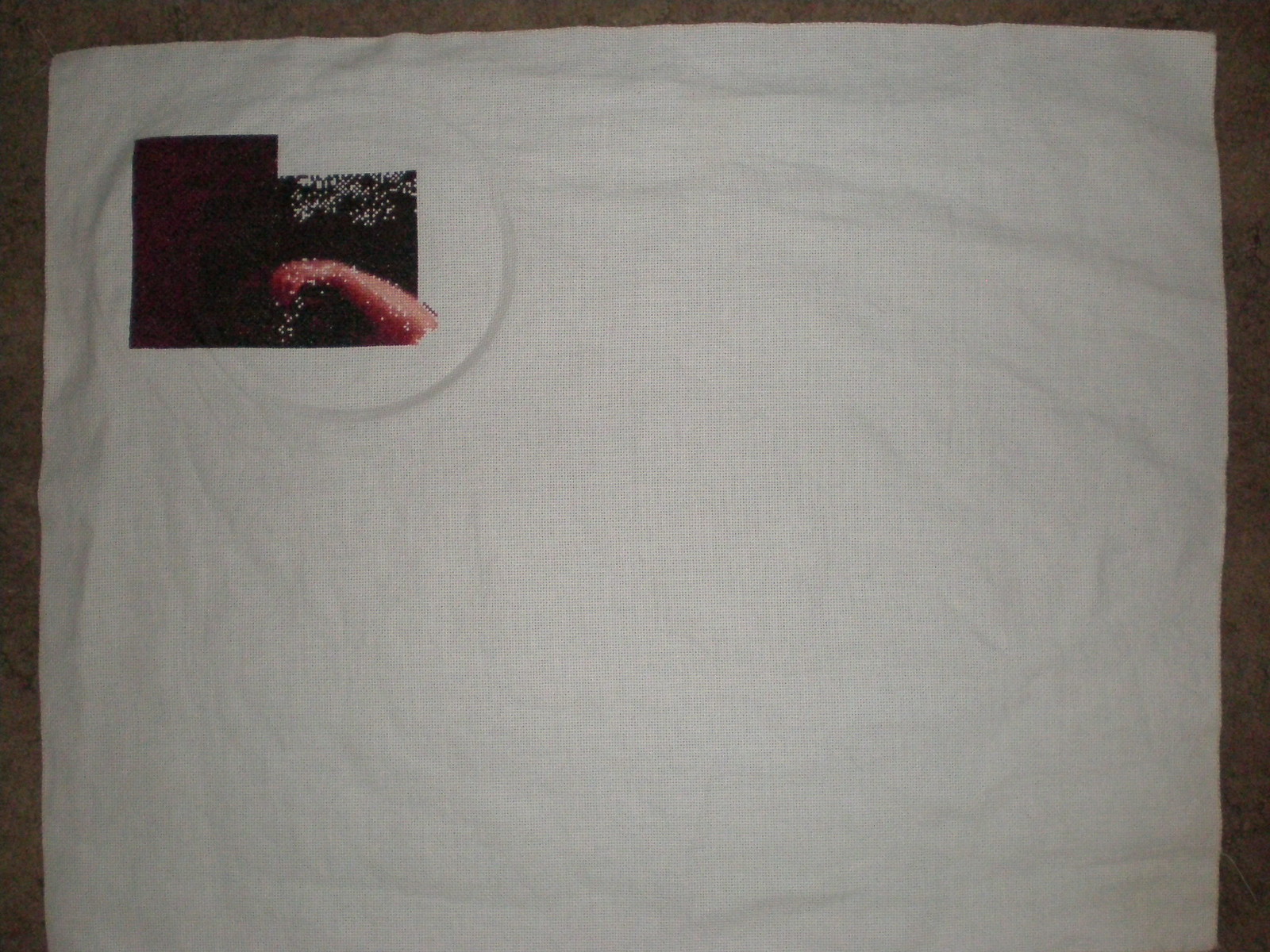This image features a textured piece of cloth, with the texture running vertically across the fabric. In the upper left corner, there's a visible indentation shaped like a circle, containing a small, detailed picture. The central element within this picture displays an orangey, bumpy, arm-like structure, set against a stark black backdrop. The image within the circular indentation is divided; one side is completely black and rectangular, while the other side varies in shape and includes additional unspecified details.